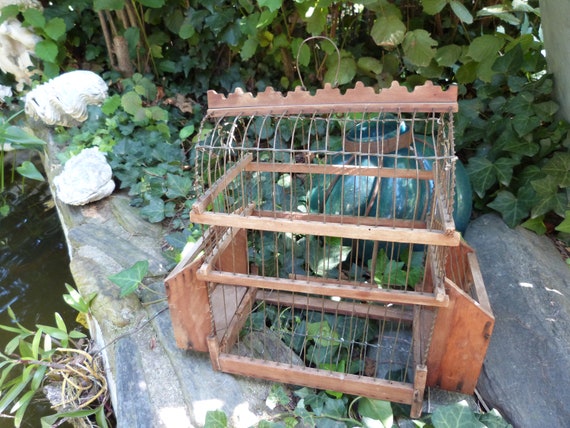This outdoor daytime photograph captures a rustic, homemade bird feeder or cage made of wire and wood, resting on what looks like a weathered wooden or rocky surface near the edge of a body of water. The feeder features three wooden shelves and two pockets, with a wire hanger at the top suggesting it is meant for hanging, potentially to feed suet to birds like woodpeckers. The background is dense with leafy, vine-covered plants in varying shades of green and blue-green, creating a lush, garden-like setting. On the left, a fragment of water peeks beneath the surface, indicating proximity to a body of water, possibly a dock. Several light-colored stones, approximately the size of fists, and an ornamental object, possibly a glass or ceramic jar, are scattered nearby. Adjacent to the feeder, a lawn ornament resembling a lamp or light fixture adds a subtle decorative touch.